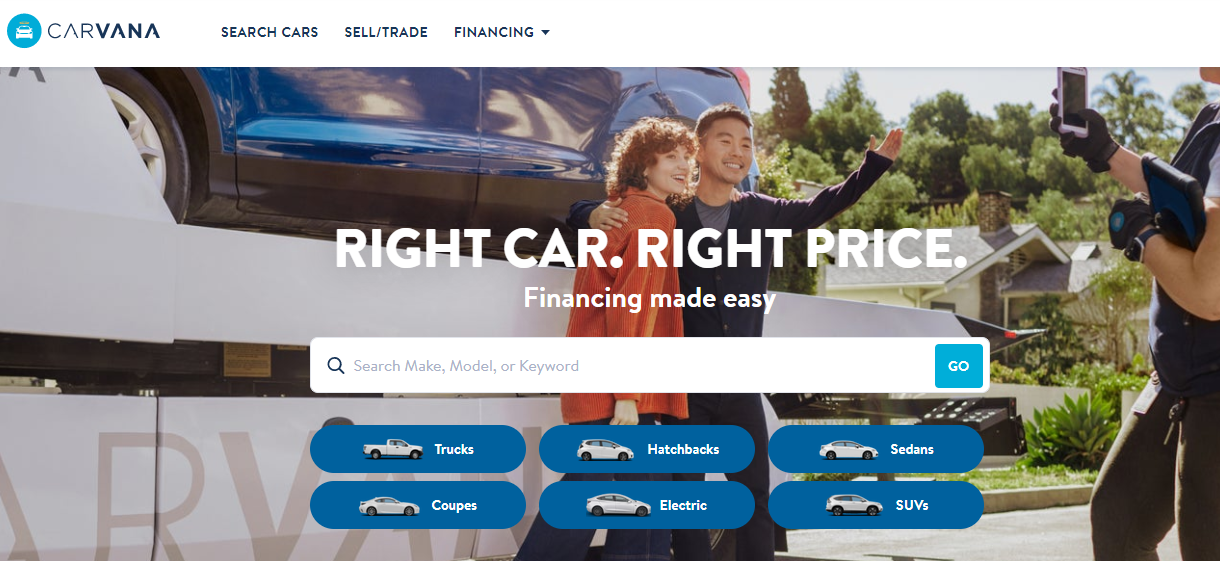This image depicts the Carvana website interface, characterized by its vibrant and appealing design. In the upper left-hand corner, the Carvana logo is prominently displayed, featuring a blue circle with a car icon. Just below the logo, navigation options include "Search Cars," "Sell/Trade," and "Financing," each accompanied by a drop-down menu.

Dominating the center of the image is a photo showing a man and a woman standing outside their home, interacting with a Carvana delivery representative. The woman, dressed in a red coat, appears to be Caucasian, while the man in a black sweater seems to be Asian. They stand in front of their house with visible neighboring homes in the backdrop. The Carvana representative, equipped with an iPad, wears black pants, a black glove, a watch, and has a Carvana badge attached. He is in the process of taking a photo of the couple, possibly documenting the car delivery process.

In the foreground of the website, a slogan reads "Right Car, Right Price, Financing Made Easy," accompanied by a search bar featuring a blue "Go" button. Below the search bar are clickable bubbles for various car categories, including Trucks, Coupes, Hatchbacks, Electric, Sedans, and SUVs. The delivery vehicle, which likely brought the new car to the couple, has the Carvana branding prominently displayed on its side. The overall layout of the website is user-friendly, emphasizing an efficient and pleasant car-buying experience.